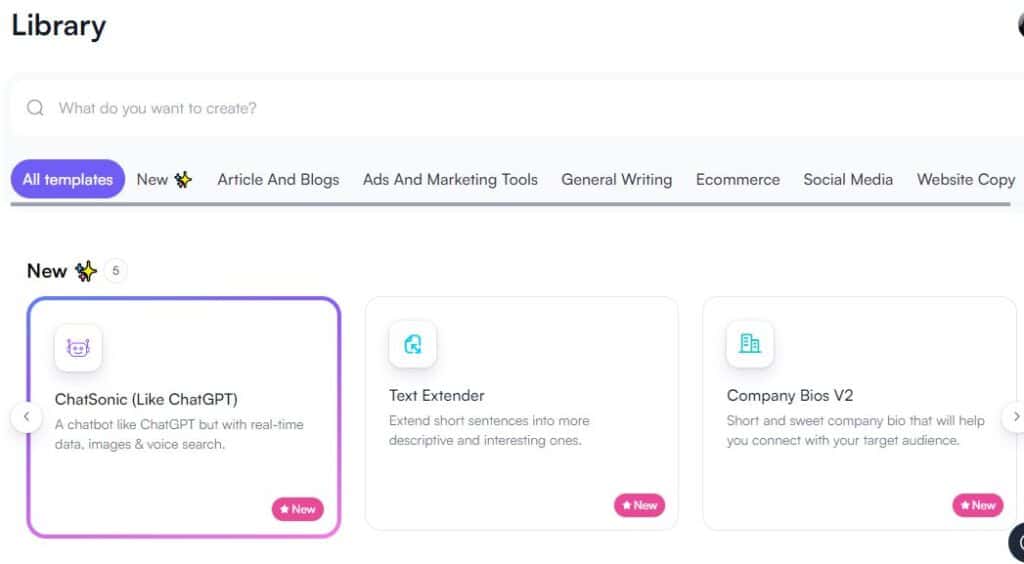The image displays a section of a website labeled "Library." At the top of this section, there's a prompt that reads, "What do you want to create?" accompanied by a search bar where users can type in their queries. Below the search bar is a list of categories: "All Templates," "New," "Articles and Blogs," "Ads and Marketing Tools," "General Writing," "E-commerce," "Social Media," and "Website Copy."

Further down, there's a highlighted section titled "New," marked with a star and the number five, indicating five new items. Three items are visible in this section, and navigation arrows on the left and right sides allow for horizontal scrolling.

At the top of the newly added items, there's a tab labeled "Chat Sonic," described as similar to ChatGPT, featuring an icon resembling an alien head within a white box. This tab is currently selected, indicated by a vibrant border in purple, royal blue, and pink, and a "New" button at the bottom.

Next to "Chat Sonic," there are two more tabs: "Text Extender" in the center and "Company Bias V2" on the right, each also marked with a "New" button at the bottom.